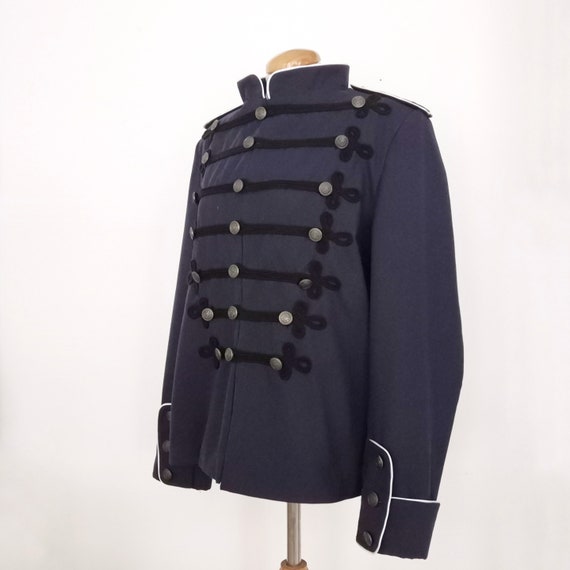The photograph, taken indoors, features a square image approximately four inches by four inches with a very pale pink background. At the center, an old-school military-style uniform jacket is displayed on a mannequin. The jacket, facing slightly to the left, is a dark bluish-gray or navy blue color. It has a high standing collar adorned with white piping, which also outlines the cuffs of the sleeves and other borders of the coat. Black braids with intricate loops extend across the chest, fastened with small round silver buttons at the left, center, and right sides of each braid. The front of the jacket is embellished with numerous buttons—approximately 21—tied together with thick black strings. The sleeves feature additional detailing with three silver buttons on each cuff. The mannequin's wooden top supports the jacket, making it appear as if it is being worn. The overall image presents the jacket against a pale backdrop, highlighting the detailed craftsmanship and historical design of the uniform coat.